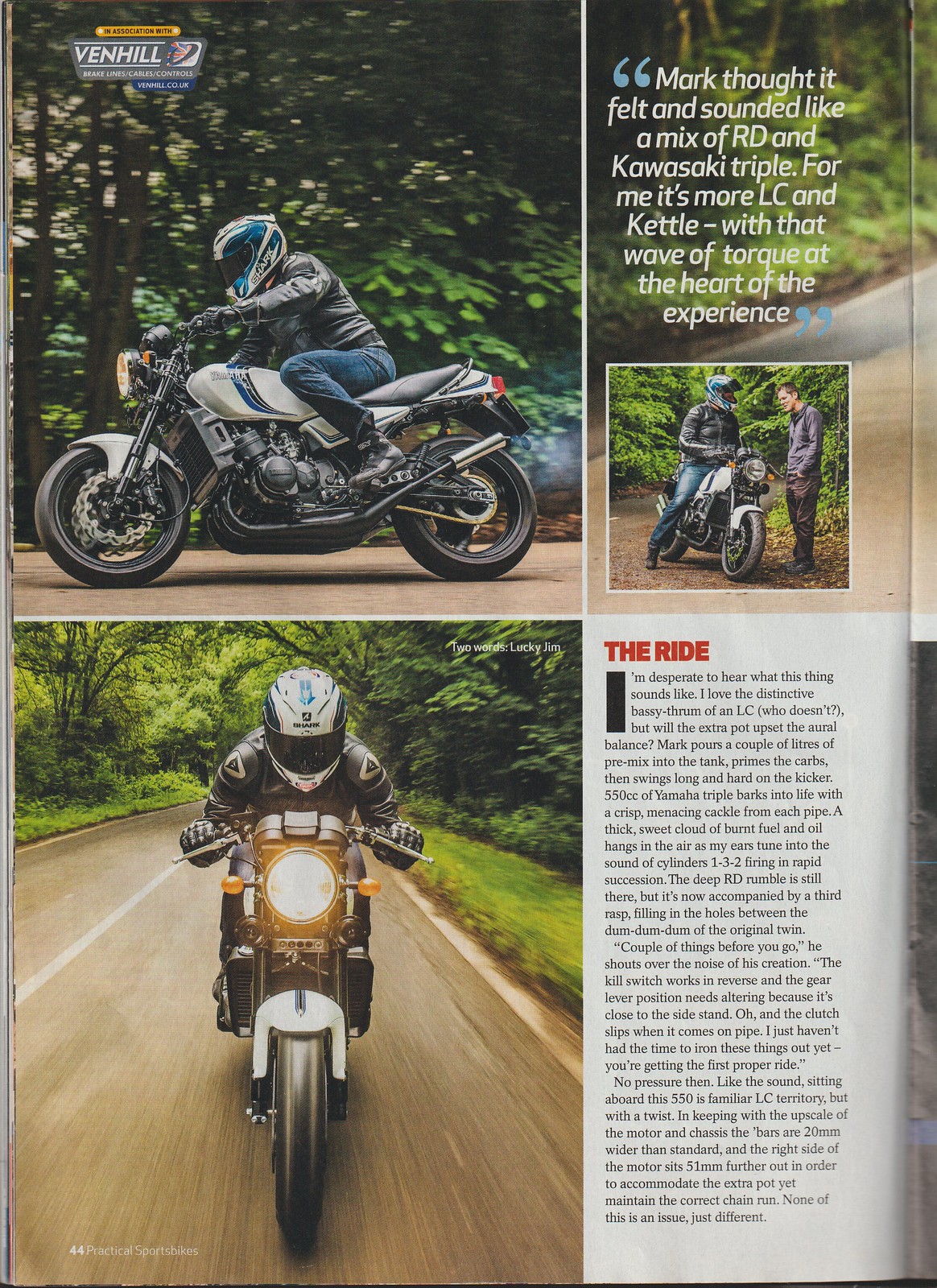The image captures the left page of a motorcycle magazine spread, featuring a collage of photographs and text. Dominating the upper left quadrant is a dynamic shot of a silver and black motorcycle leaning right, roaring down a tree-lined road with exhaust smoke billowing behind. The rider is clad in blue jeans, a black leather jacket, and a blue, black, and white helmet. Above this image, the Venhill logo and the tagline “brake lines, cables, controls, venhill.co.uk” are prominently displayed.

Beneath this, the lower left quadrant presents the same motorcycle barreling directly towards the viewer, headlight blazing and the road a blur beneath, framed by a canopy of trees. The helmet bears the "Shark" brand, indicative of its robust design. 

Adjacent to this, in the upper right quadrant, there’s a quote against a forested backdrop: "Mark thought it felt and sounded like a mix of RD and Kawasaki Triple. For me, it's more LC and Kettle with that wave of torque at the heart of the experience." Below this quote, there's another image showing a man talking to a rider who sits stationary on the motorcycle, underlining the hands-on, experiential nature of motorcycle enthusiasts.

The lower right section of the page is filled with a dense, descriptive text block under the red-lettered heading "The Ride." This narrative immerses the reader in a vivid depiction of the motorcycle's performance, the rider’s experience, and the intricacies of the bike’s design and modifications.

With a palette of green, white, black, red, and blue, this magazine page captures the essence of motorcycling culture with its rich imagery and detailed recounting of the rider's journey and the motorcycle's capabilities.